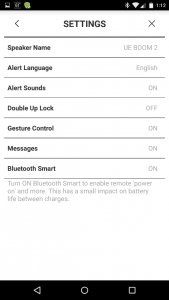The image depicts a cell phone settings screen with a notably poor resolution. At the top of the screen, there's a black bar displaying several icons. From left to right, these icons include Bluetooth, Wi-Fi, cellular signal bars, a full battery, and the current time in the p.m., although the exact time is not clear. Below this bar, on a white background, is a user interface layout featuring various settings options.

At the top center of the white background is a left-pointing arrow on the left side, "Settings" in the middle, and an "X" on the right, followed by a dividing line. 

Several settings options are listed below this line:
- "Speaker Name" on the left with "UE Boom 2" on the right.
- "Alert Language" on the left with "English" on the right.
- "Alert Sounds" on the left with "On" on the right.
- "Double-Up Lock" on the left with "Off" on the right.
- "Gesture Control" on the left with "On" on the right.
- "Messages" on the left with "On" on the right.
- "Bluetooth Smart" on the left with "On" on the right.

Below the Bluetooth Smart setting, a note states: "Turn on Bluetooth Smart to enable remote power on and more. This has a small impact on battery life between charges."

At the bottom of the screen, there's additional white space followed by a black navigation bar with three icons: a left-pointing arrow, a circle, and a square. A partially visible green icon is present in the upper left corner of the status bar, the specific details of which are not discernible. The predominant colors on the screen are black, white, green, and gray.